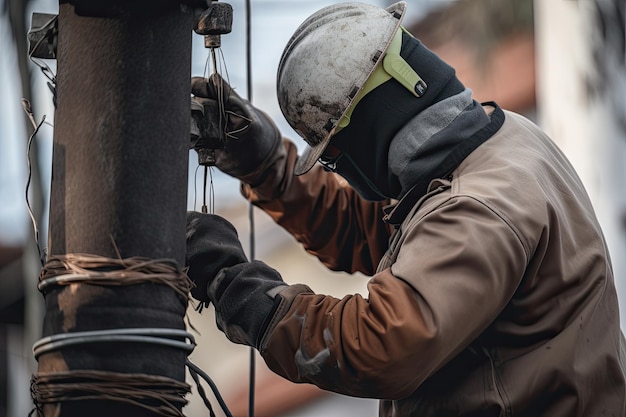This image depicts a heavily protected power line worker or electrician intently repairing some wiring on an electrical pole. The worker is standing on the right side of the image, dressed in a thick brown jacket that transitions to an orangish hue near the sleeves, and is equipped with black rubber gloves. He is wearing a white hard hat with a bright yellow strap that is unattached at the left ear, and his face is mostly covered by a dark gray protective fabric, complemented by protective eyewear. The worker is extending his left arm towards the pole, manipulating thin wires connected to the structure. The pole, which stands on the left and appears dark brown and rusty, supports three distinct sets of wires wrapped horizontally around its base. The lowest set of wires is copper colored, followed by a set of silver wires, and above that, another set of copper wires. The man’s intensive focus is evident as he looks down at the intricate wiring, ensuring precise work on the electrical project.